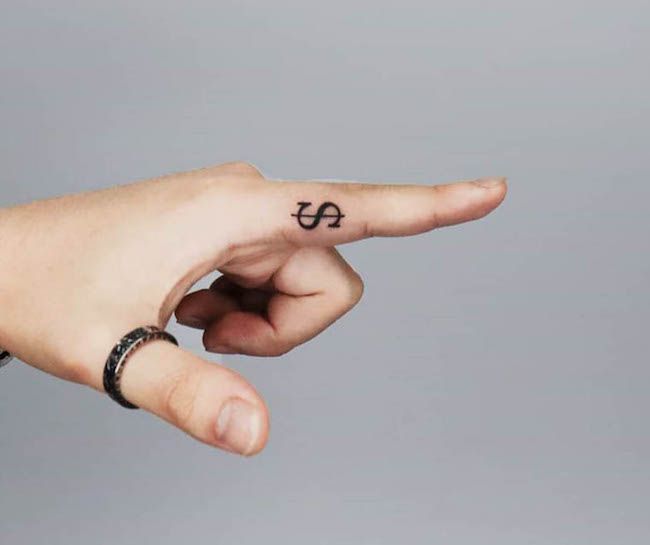This photograph features a close-up of a Caucasian left hand set against a gray background. The hand is captured in a pointing gesture, with the index finger extended horizontally from left to right and the thumb somewhat extended outward. Notably, the index finger, which is pointing directly outward, is adorned with a black tattoo of a dollar sign ($). Additionally, the thumb bears a dark-colored ring with silver accents. The image is cropped at the wrist, focusing exclusively on the hand and its distinctive markings. While the exact meaning behind the pointing gesture and the dollar sign remains open to interpretation, they are the central elements of this minimalist composition.